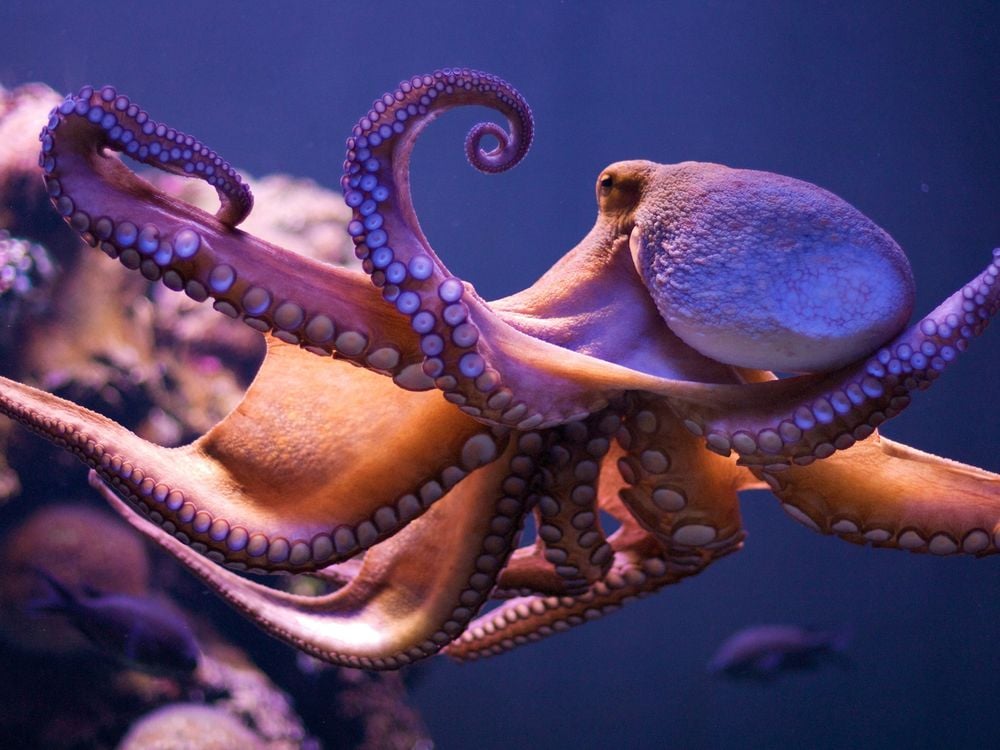The photograph showcases a mesmerizing underwater scene or possibly an aquarium, dominated by a horizontally-oriented rectangular frame with an immersive deep blue, almost indigo, backdrop. The central focus is a striking close-up of an octopus, whose head occupies the right side of the image. The head is textured with several wrinkles and features a notable crater-like indent. The octopus, exhibiting a harmonious blend of purplish-pink to orange-yellow hues, stretches its eight tentacles in various directions, each adorned with white suction cups bordered by purple circles.

Near the octopus's head, a lump indicates the position of its eye, enhancing its distinctive form. In the bottom right, the image hints at another sea creature, possibly a crab, whereas a prominent rock formation on the left is adorned with colorful marine plants. The rocks display shades of pink, brown, and tan, contributing to the vibrant underwater ecosystem. Additionally, blurry coral structures and tropical fish, tinted in purplish colors, swim gracefully in the background, complementing the octopus and creating a lively, captivating underwater tableau.